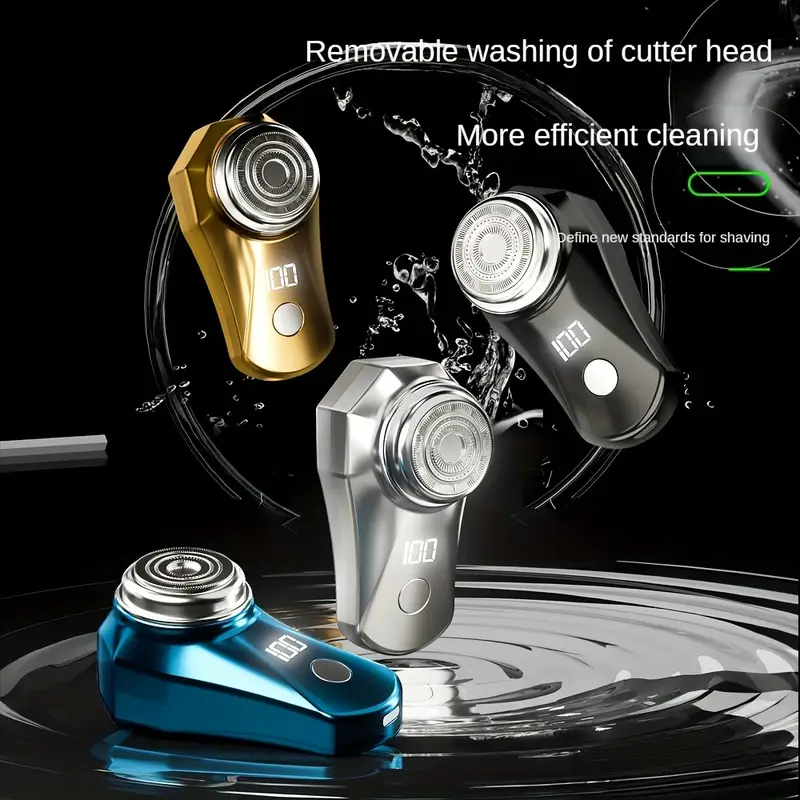The advertisement showcases four cordless electric shavers set against a sleek black background, emphasizing their modern and efficient design. Each shaver is showcased in a distinct, vibrant color: neon electric blue, metallic silver, charcoal gray, and metallic gold. The shavers are positioned artfully, with the blue one laying down, the silver one standing upright on its end, the gold one floating in the upper left, and the black one floating to the right of the silver shaver.

In the upper right corner, the text "Removable Washing of Cutter Head," "More Efficient Cleaning," and "Define New Standards for Shaving" is displayed in white, reinforcing the product's innovative features. The shavers each feature a digital display reading "100."

Adding to the dynamic composition, rippling water effects surround the standing and floating shavers, with water droplets and splash patterns indicating that the shaver heads are designed to be washable, enhancing the usability and hygiene of the product. The overall aesthetic conveys cleanliness, efficiency, and modernity.